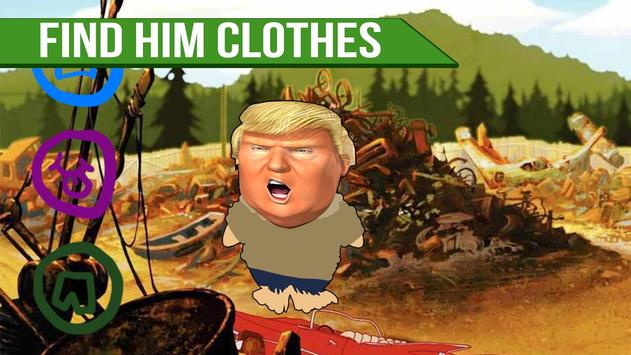The image depicts a cartoon-styled character with Donald Trump's face superimposed onto it, standing at the center of a junkyard scene. The surroundings are cluttered with a pile of assorted trash, including an old car, a broken plane, and a boat. In the background, there are trees and various discarded items forming a collage. The character has an exaggerated square jaw, orange-toned face, and yellowish-blond hair. He wears a tattered, brownish-beige t-shirt and his oddly round, apparently amputated arms lack hands, while his feet are shapeless blobs. In the top left corner of the image, a green ribbon with white text reads, "Find him clothes." Nearby, some hand-drawn labels in shades of blue, purple, and green are visible. The overall style of the image suggests it might be a screenshot from a low-budget flash game or a meme with a cartoon aesthetic.